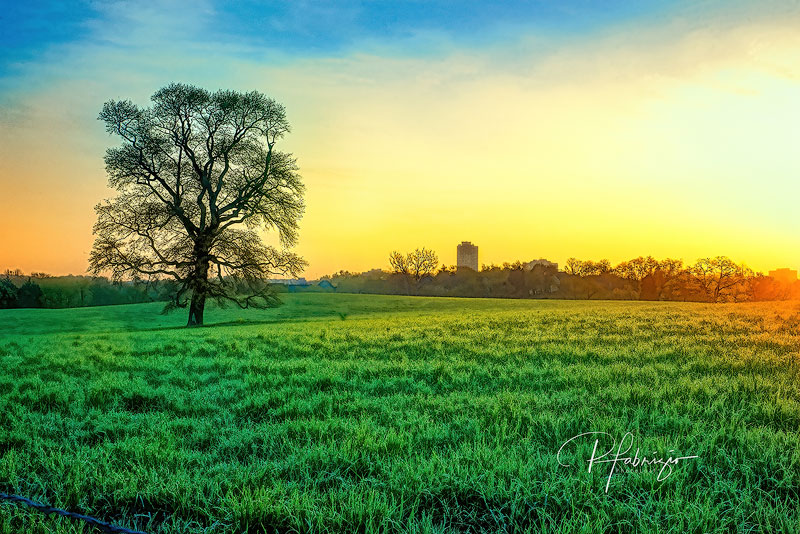The image is a vibrant and artistic representation of a solitary, large tree standing leafless in the middle of an expansive grass field. The grass is a bright, vibrant green, dominating most of the foreground and giving way to a slight, rolling hill. The tree is positioned off-center to the left, appearing somewhat lonely and stark against the spacious landscape. In the far distance, a hint of more trees and a building are barely visible, adding depth to the scene. The setting sun casts an orange and yellowish glow over the field, contrasting with the blue at the top of the sky. The artist's signature is subtly placed in the bottom right, completing this striking, picturesque scene.